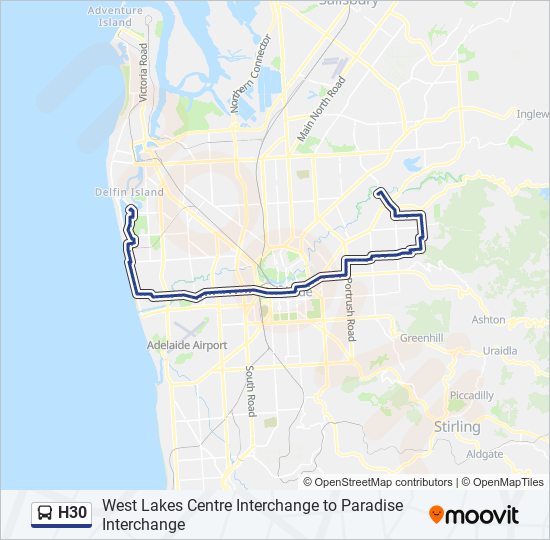A detailed screenshot of a map is displayed, taken from the Moveit application, spelling M-O-O-V-I-T, a navigation service. The depicted map centers around Adelaide, Australia, verified by the presence of notable locations such as Adelaide Airport and Stirling. The map outlines a route between West Lakes Centre Interchange and Paradise Interchange, marked with the highway identifier H-30. The path is highlighted in blue, tracing the journey from point A to point B. It ultimately ends near Delphin Island, located on the coastal waters. In addition, Adventure Island is marked near the top of the map. The map’s color scheme includes muted greens for the land and blue for the water bodies. The GPS icon and Moveit logo are also present beneath the map, enhancing the navigational details.